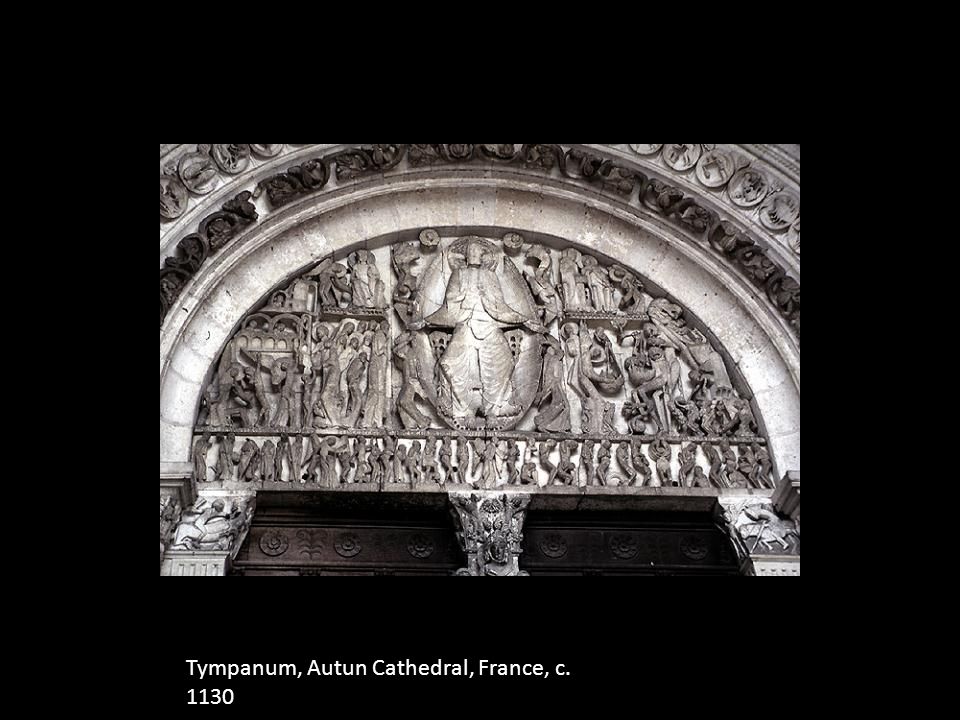This black-and-white photograph depicts an intricately carved stone tympanum from the Autumn Cathedral in France, dating from around 1130. The stone mural spans above the doorway, supported by engraved columns adorned with figures of people, possibly riding horses. The central figure dominating the composition extends their arms outward, flanked by what appears to be a halo, suggesting a divine or god-like presence. Surrounding this figure are countless smaller figures, engaged in various activities, forming a detailed and dense scene. The text beneath the image reads "Tympanum, Autun Cathedral, France, c. 1130," confirming its historical and geographical context.